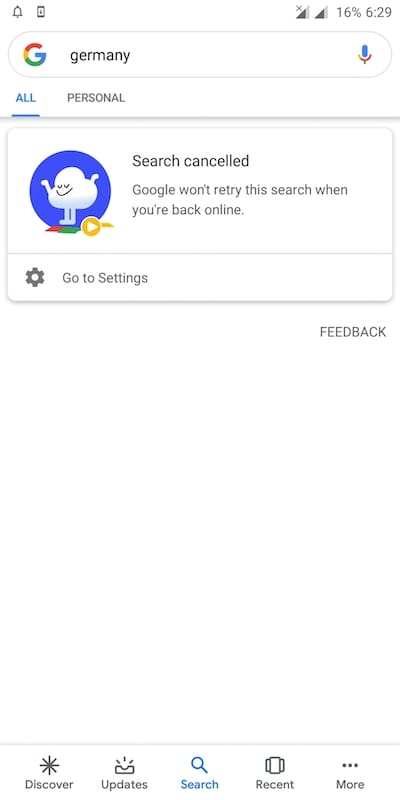A screenshot captures a smartphone screen displaying the Google Search app in action. At the top of the screen, the familiar Google search bar is visible, featuring the iconic 'G' logo on the left. Adjacent to the logo is the search input field, allowing users to type in their queries, and a microphone icon on the right for voice-activated searches. The user has searched for "Germany," but an auto-response message appears below with an icon of a cloud displaying a shrugging gesture. The message reads, "Search canceled. Google won't retry this search when you're back online," indicating that the search was aborted. Beneath this notification is an option labeled "Go to settings." At the very bottom of the screen, a navigation bar is present with multiple options: Discover, Updates, Search (which is currently highlighted), Recents, and More. This detailed layout confirms that the user was utilizing the Google Search app to look up information about Germany but opted to cancel the search before it could be completed.